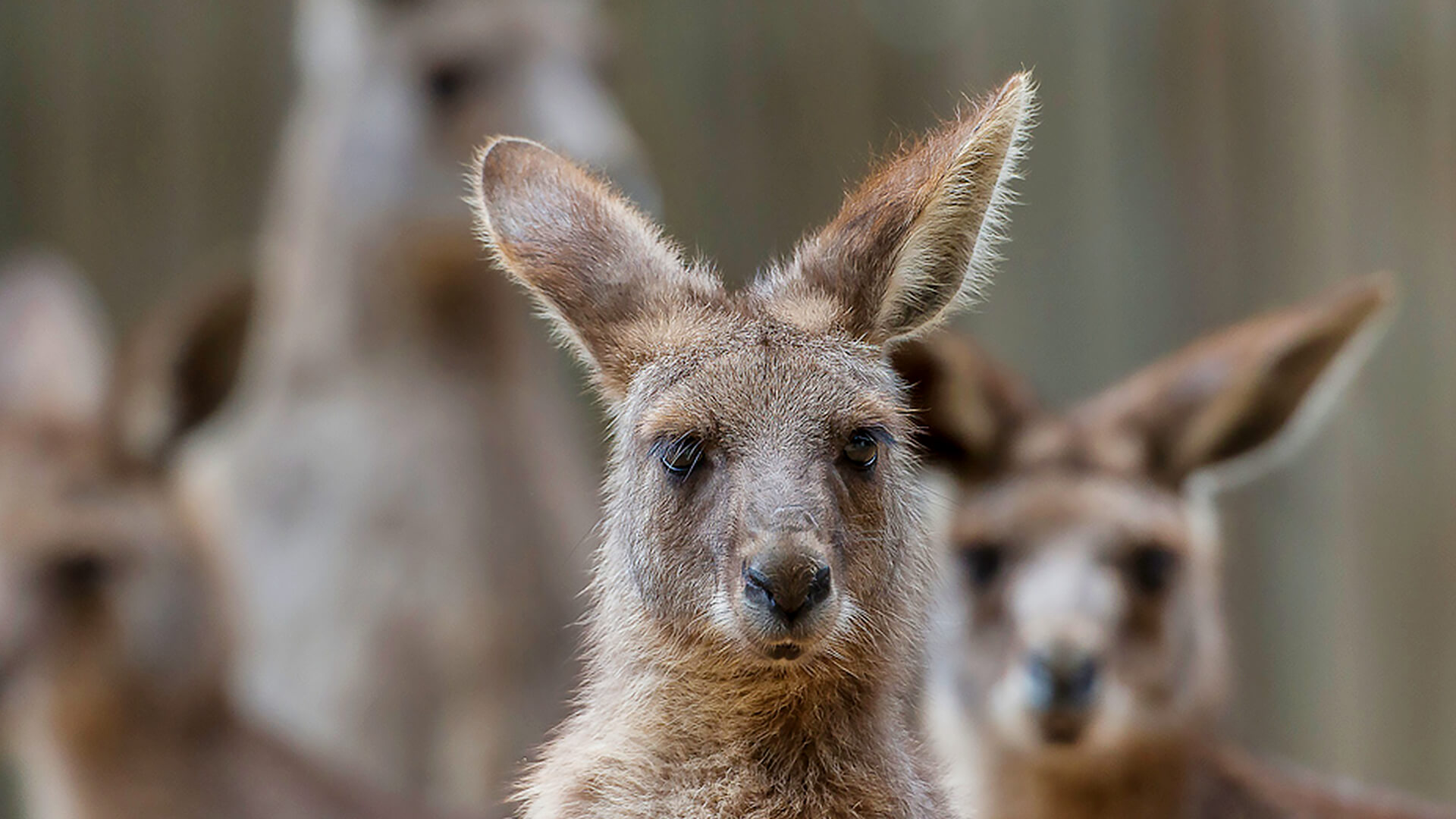The photograph captures a juvenile kangaroo standing prominently in a natural setting. The young kangaroo, positioned in the foreground, faces the camera with its ears perked up in a distinct V-shape. Its fur showcases a range of brown shades, with a light brown neck and medium brown face adorned with hazel eyes, black eyelashes, and a dark nose. Fine details are visible, especially the delicate fur on its ears, which are light brown inside and medium brown outside. In the background, three more kangaroos are visible, though they are significantly blurred and lack the sharp detail of the central subject. The largest among these, to the left, and others scattered behind, are nearly indiscernible due to the image's focus on the young kangaroo in the foreground.